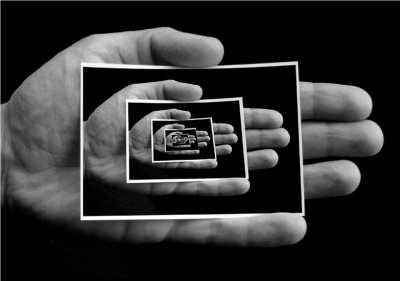The grayscale image showcases an optical illusion featuring a left hand with extended fingers, positioned against a stark black background. The hand, of grayish complexion suggesting a monochrome treatment, holds a photograph exhibiting the very same image. This recursive effect continues, with each iteration of the hand holding a photo shrinking progressively towards the center, creating a visual tunnel that seemingly extends into infinity. Each photo within the photo is framed by a thin white border, contributing to the repetitive and endless loop illusion. The photograph highlights the intricate details of the hand's texture and shape, complete with visible fingers and a slightly wrinkled appearance, further emphasizing the artistic, infinite regression theme.